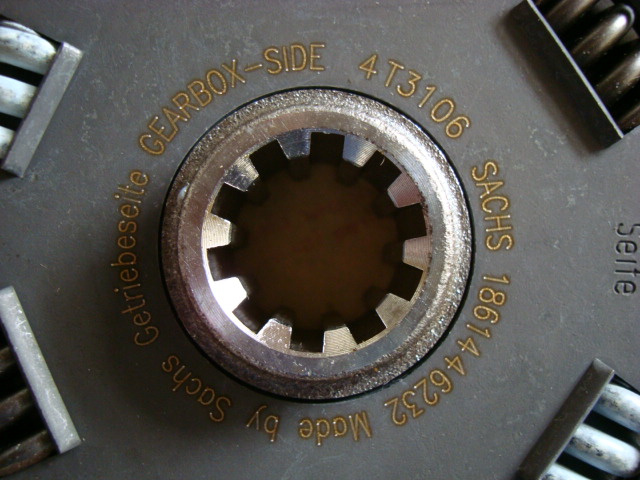This detailed photograph is a close-up of what appears to be a clutch plate for an automobile. The central feature is a chrome circular component with cogs designed to fit a shaft. Surrounding the middle are four corners equipped with springs. The plate itself, predominantly gray, is embedded with various markings including "gearbox side," "4T 3106," and "186144," all indicating manufacturing details. Prominently inscribed is the name "SACHS," the manufacturer. The background is a brownish-gray metal, contrastively highlighting the intricate details of the clutch.